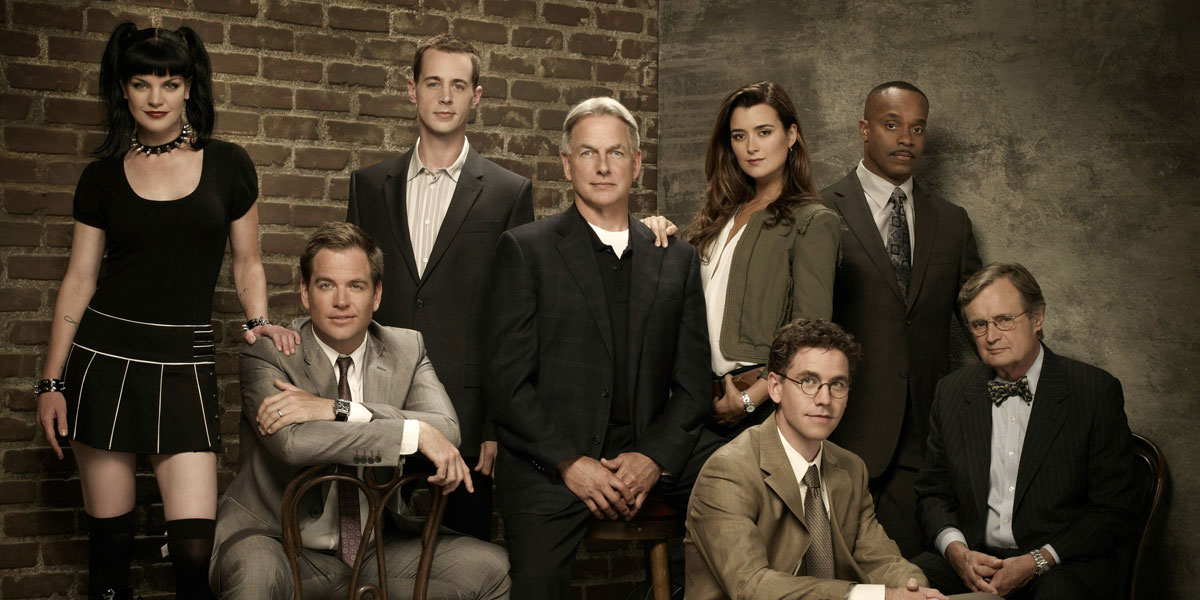The photograph is a detailed, indoor, landscape shot of a mixed-gender and interracial cast from a television show featuring actor Mark Harmon, who stands centrally. Mark Harmon is clad in a dark, checkered black suit with a black undershirt and a white T-shirt, his short gray hair neatly styled, and his hands clasped in front of him as he looks directly into the camera. Surrounding him are seven other characters:

To Mark Harmon’s immediate left (our right) stands a woman with long, dark, curled hair, wearing an olive green short jacket and a white top, her hand casually resting on his shoulder.

Next to her, further to the right, is an African-American man in a dark suit, white shirt, and a dark patterned tie. To the far right, seated, is an older gentleman with wire-rimmed glasses, a spotted bow tie, and a dark blazer; his hands are also clasped together.

In front of the older gentleman, another man is partially visible, showing only his upper torso. He sports a very light brown suit, a light brown tie, a white shirt, short curly hair, and round-rimmed glasses.

To the left of Mark Harmon (our left), begins with a man standing in a dark suit coat with a white collared shirt. He has short dark hair and no tie, and is looking directly at the camera. Beside him, sitting backwards on a chair is a man wearing a light gray suit, white shirt, and brown tie, arms folded on the back of the chair, exhibiting short brown hair.

At the far left is a woman in a short, black, scoop-necked dress with white stripes, long stockings, knee-high boots, and a spiked choker necklace around her neck. She wears heavy makeup with bright red lips and dark eyeshadow, her black hair styled into pigtails, and she rests one hand on the seated man's shoulder.

The background behind the group transitions from light orange bricks on the left to a gray backdrop on the right, adding texture to the formal and coordinated ensemble.